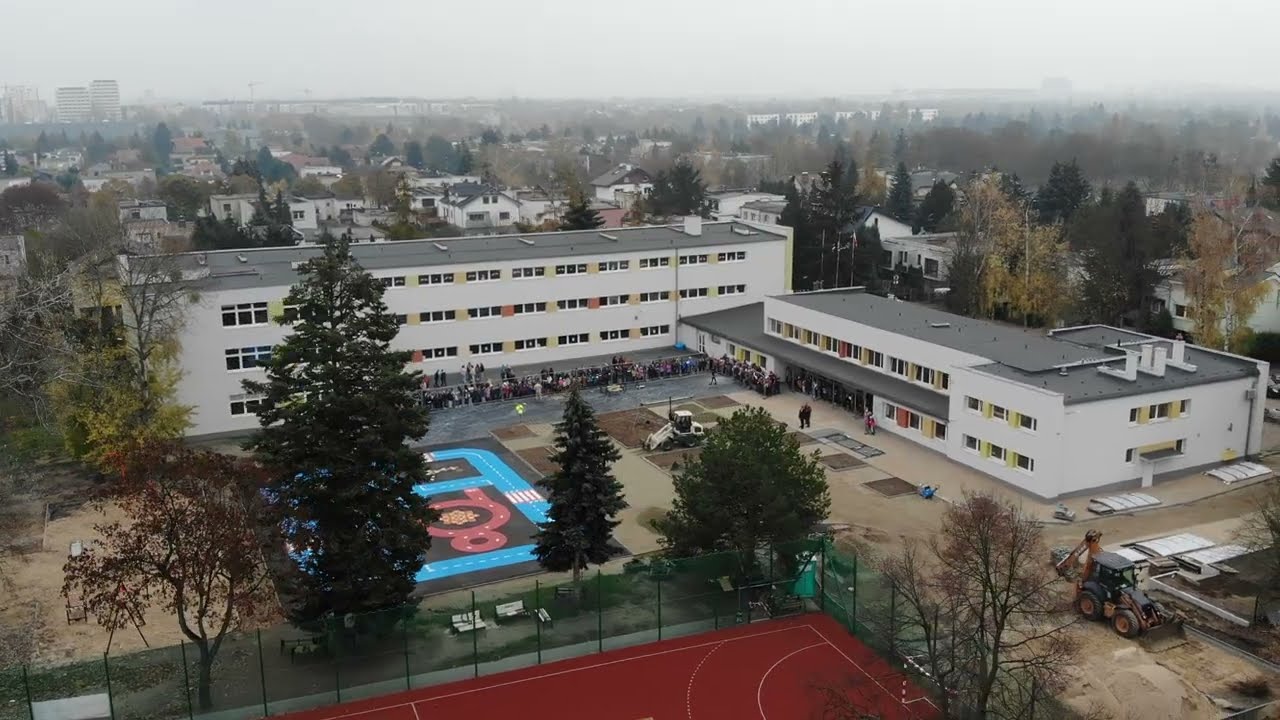The aerial image depicts an institutional L-shaped complex, likely a college, consisting of two prominent white buildings with varying levels—one with two stories and the other with three. Both structures have rows of windows. The buildings are surrounded by numerous trees and are positioned close to each other. In the foreground of the image, there is a red basketball court, and in the distance, a track or course outlined in blue and red can be seen. A large crowd of people is lined up in an L-shape along the exterior of the buildings. Additionally, there is construction equipment, including a backhoe, to the right side of the image. Behind the primary buildings, various other structures and houses are visible, along with more trees interspersed throughout the area. The overhead perspective, likely taken by a drone, also captures a strip of gray sky at the top of the image.